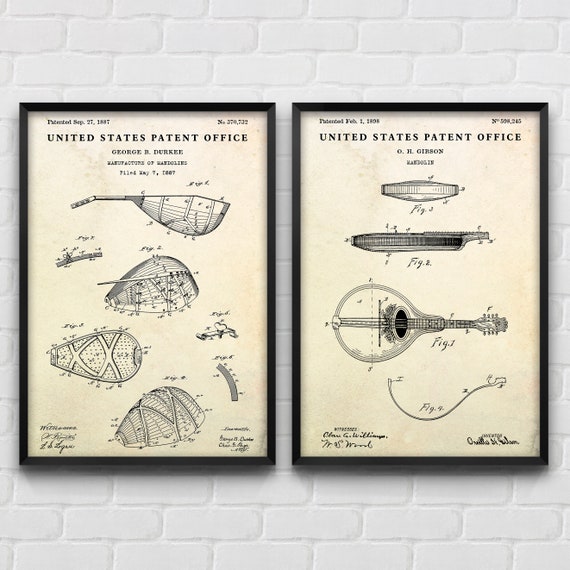The photograph features two framed pages of an antique patent, both mounted on a digitally rendered white brick wall. These yellowed patent pages, displaying signs of age, are encased in sleek black frames. The page on the left prominently reads "United States Patent Office" in bold, and although the exact date is hard to discern, it seems to be patented on September 27th, 1887, by George B. Durkee. This page illustrates detailed diagrams of a mandolin, showcasing its internal and external construction from various angles. The page on the right contains similar patent details, suggesting it's filed by O. H. Gibson, and features additional views of a mandolin, possibly indicating a different aspect of the instrument’s design. Each page is densely packed with technical drawings marked with figure numbers and accompanied by text too minute to discern clearly, potentially including specifications, measurements, and signatures. The white brick wall backdrop contrasts with the sepia-toned parchment, highlighting the historical significance of the patents.